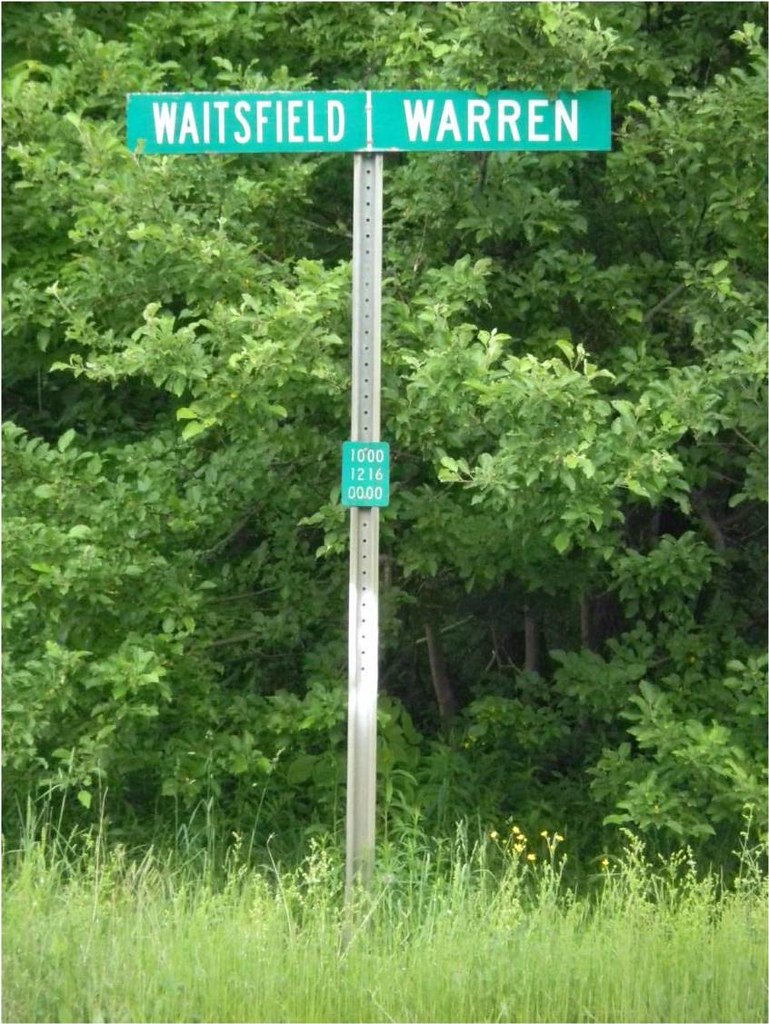This photograph, taken in a rural area during daytime, captures a green street sign mounted on a gray metal post. The sign sits at the top of the post, perpendicular, forming a T-shape. The background of the rectangular sign is dark green, featuring white capital letters spelling "Waitsfield" on the left and "Warren" on the right, separated by a vertical white line. Below this primary sign, about midway down the post, there is a smaller rectangular green sign with three lines of white numbers: "1000," "1216," and "0000". At the bottom edge of the image, unkempt, long grass with shades of light and dark green and specks of yellow is visible. The background is filled with dense tree canopy, showcasing an array of branches and leaves in various shades of green, which extends out of the frame, emphasizing the secluded nature of the location.